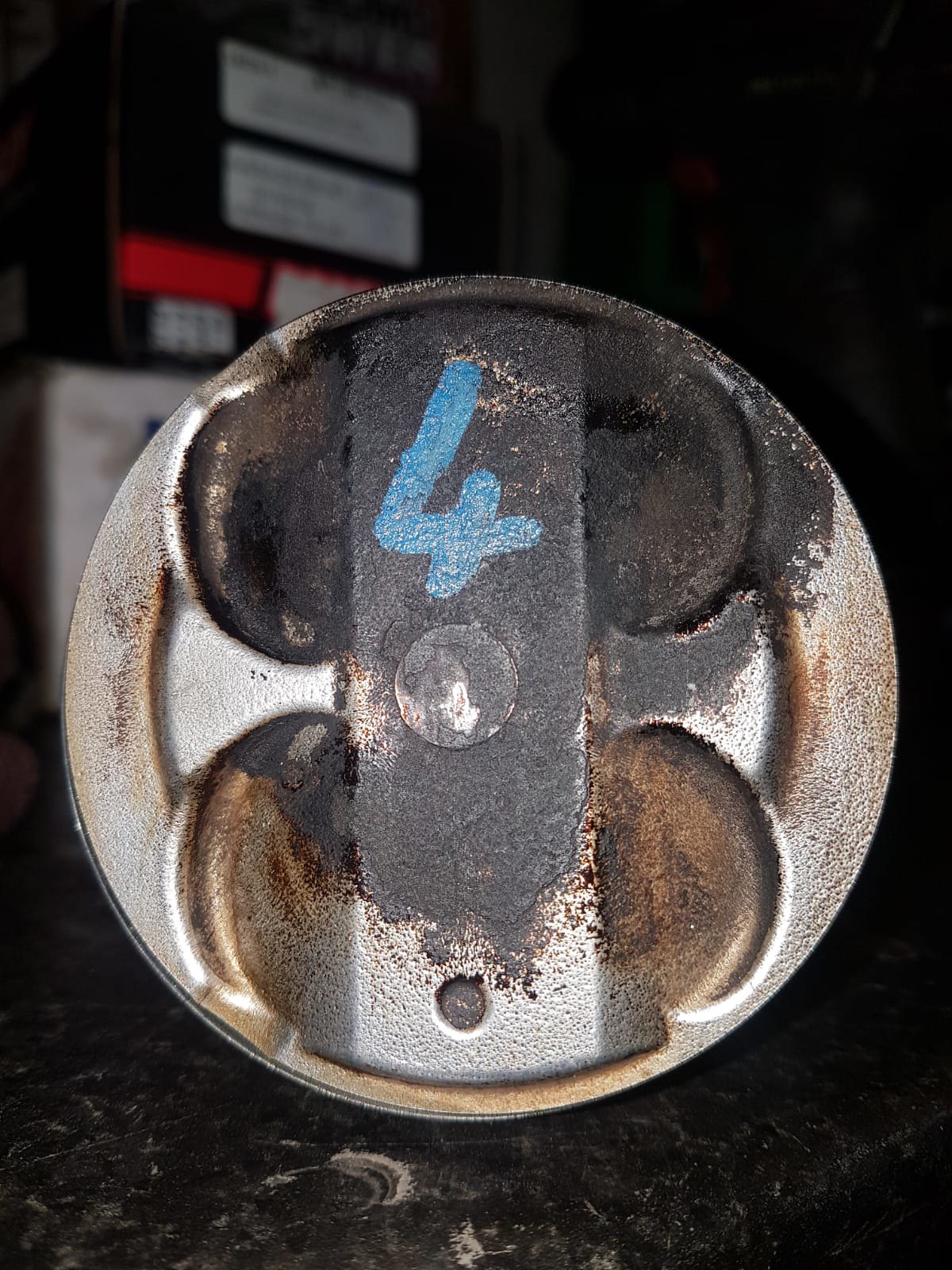This color photograph, taken indoors, captures a close-up of a rusted, cylindrical object lying on a black marble table. The object, which resembles a bolt or cylinder, has four indentations positioned at 11, 2, 5, and 7 o'clock on its bottom part. Notably, the silver base transitions into a burnt or blackened upper section, covering approximately two-thirds of its length. Prominently featured on the rusted surface is the blue number “4,” appearing both stamped and painted onto the metal. 

In the background, the room is dimly lit, revealing a bulletin board with indistinct white and red rectangles, likely containing text but blurred beyond legibility. Additionally, a shelf to the left holds black boxes with white labels, possibly batteries. The overall scene combines elements of industrial decay and minimalistic interior details.